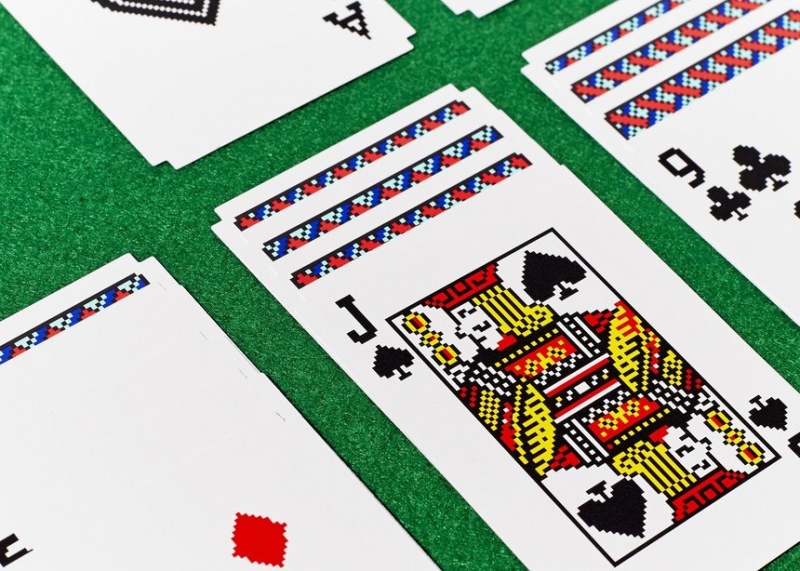The image is a close-up shot of three piles of playing cards, arranged diagonally with the top edges pointing toward the upper left corner and the bottom edges toward the lower right. At the center of the composition is a Jack of Spades on top of three face-down cards, which have a distinctive red and blue "V" pattern across their backs. To the right, partially visible in the upper right corner, is another stack of three cards, with the upper left corner of a Nine of Clubs peeking out. In the bottom left corner, there is a face-up card showing a red diamond near its edge, sitting above one face-down card. Toward the upper left, extending to the middle of the image, an Ace card lies face-up, though its suit is obscured. The cards are laid out on a textured green surface. The lines and details of the cards exhibit a pixelated quality, giving them a jagged, digital appearance.